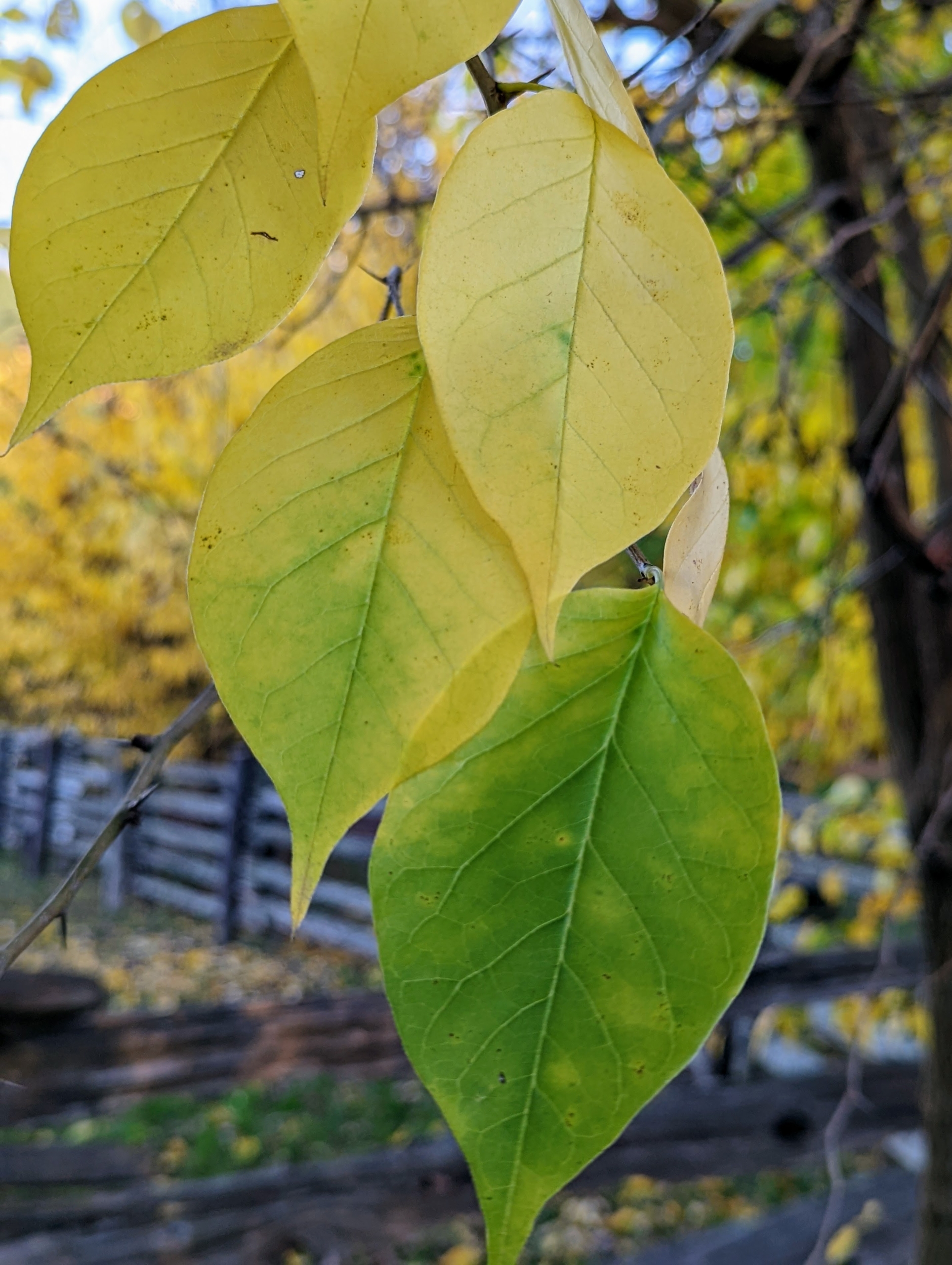This photo captures a detailed close-up of a tree branch with four prominently featured leaves. The leaves display a transition in color from green to a cheerful yellow, indicative of the fall season. The most vivid green leaf is situated near the bottom-middle of the image, with its color lightening to yellow towards the top. Thin stems extend from this central green leaf, connecting it to the other leaves and ultimately to a branch that runs between them. In the background, which is skillfully blurred to emphasize the leaves in the foreground, more trees can be spotted along with a wooden fence. The daylight setting enhances the natural hues and fine details, such as the veins of the leaves, making it an evocative nature photograph.